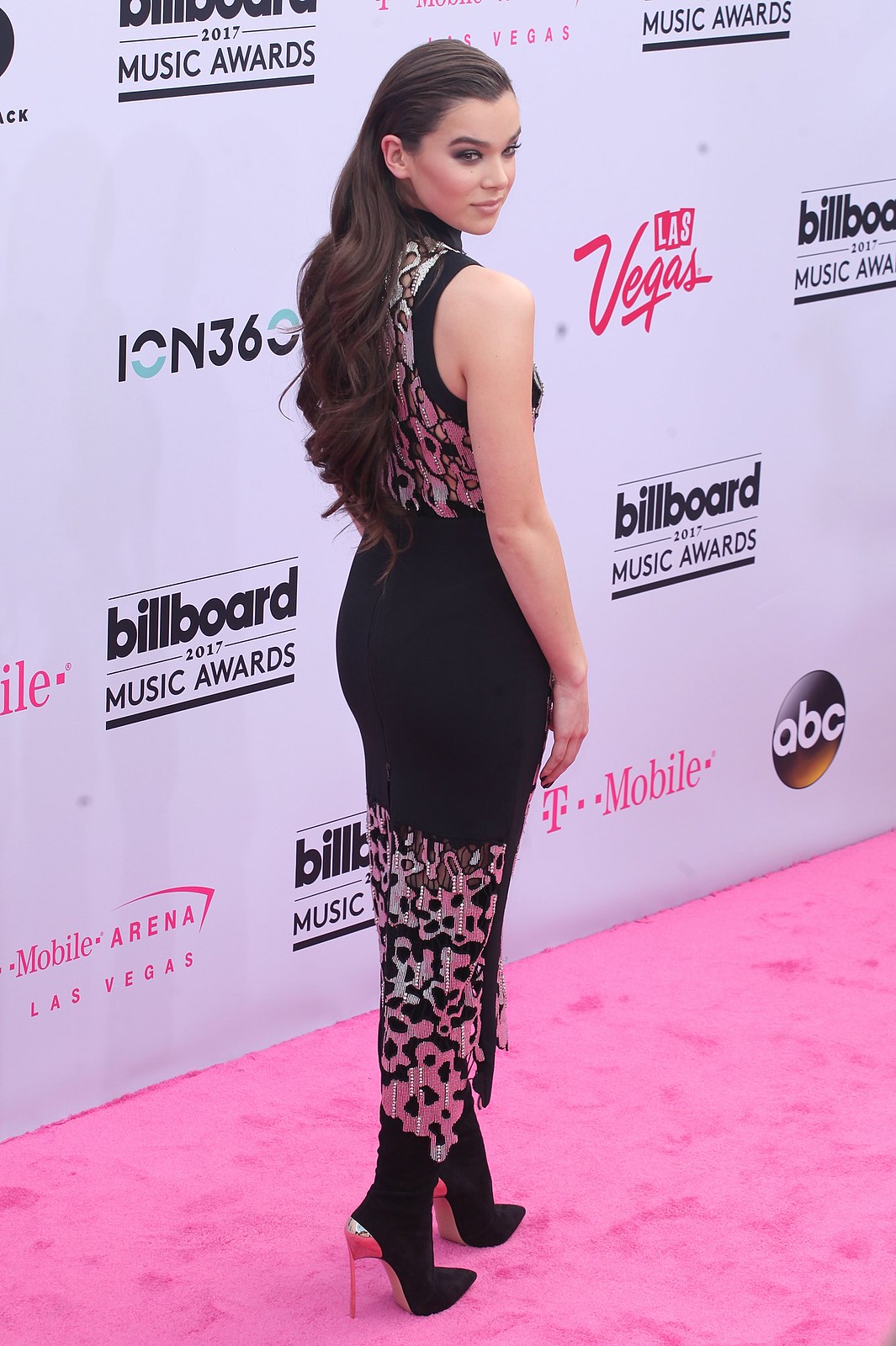In this image, actress and singer Hailee Steinfeld is captured on the pink carpet at the Billboard 2017 Music Awards held in Las Vegas. She is elegantly dressed in a striking black gown with unique design elements. The gown is form-fitting and features a pinkish floral pattern at the shoulders and thighs. Her high heels are black with eye-catching pinkish-silver heels. Hailee's long brown hair flows down her back as she looks over her shoulder, smiling at the camera. The backdrop behind her prominently displays various logos including a white Billboard 2017 Music Awards sign, a pink T-Mobile logo, and the ABC television logo in a black circle. Additional mentions of Las Vegas and ION 360 can also be seen among the advertisers.